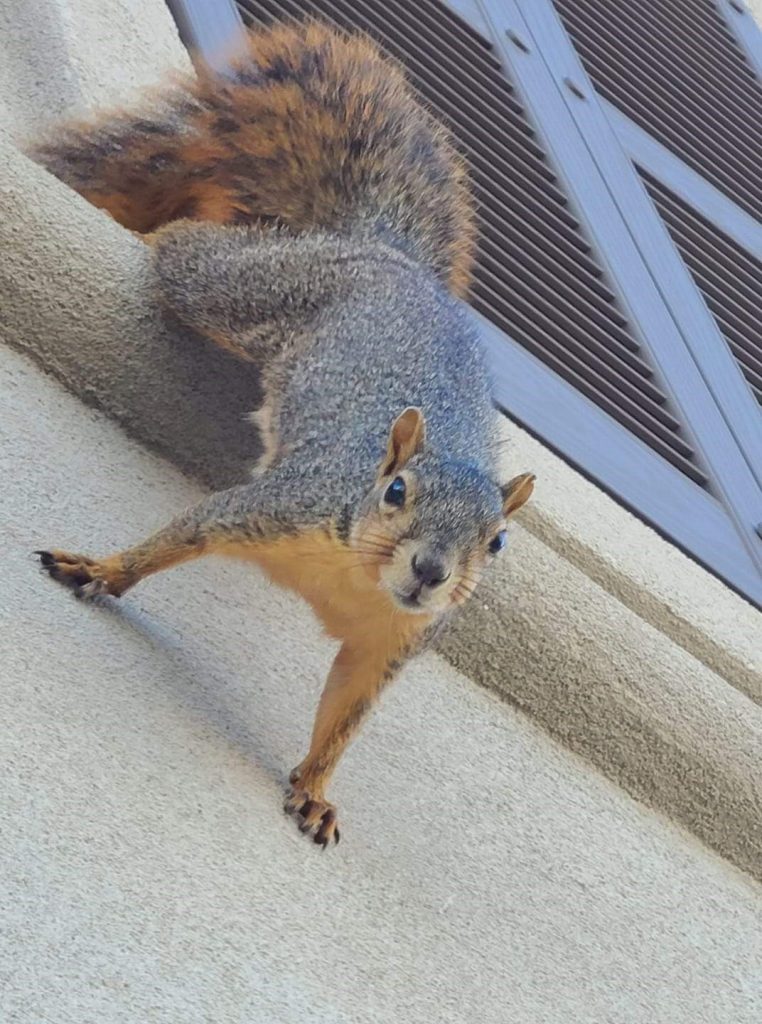This photograph captures a well-fed red squirrel, commonly referred to as a fox squirrel, in a moment of curiosity and motion. The squirrel is perched on a small curb or ledge against a light beige or grey stucco wall, its position giving the impression that it's scaling the wall. The squirrel's front paws grip this side of the curb, while its hind feet and bushy tail, which is reddish with black streaks, remain on the other side. It has a distinct coloration with a grey-brown back, beige-caramel underbelly, black claws, and beady black eyes. The squirrel is looking straight at the camera, seemingly inquisitive. In the background to the right, there is a green or brown shutter, possibly part of double wooden doors, adding a further layer of context to the outdoor setting.